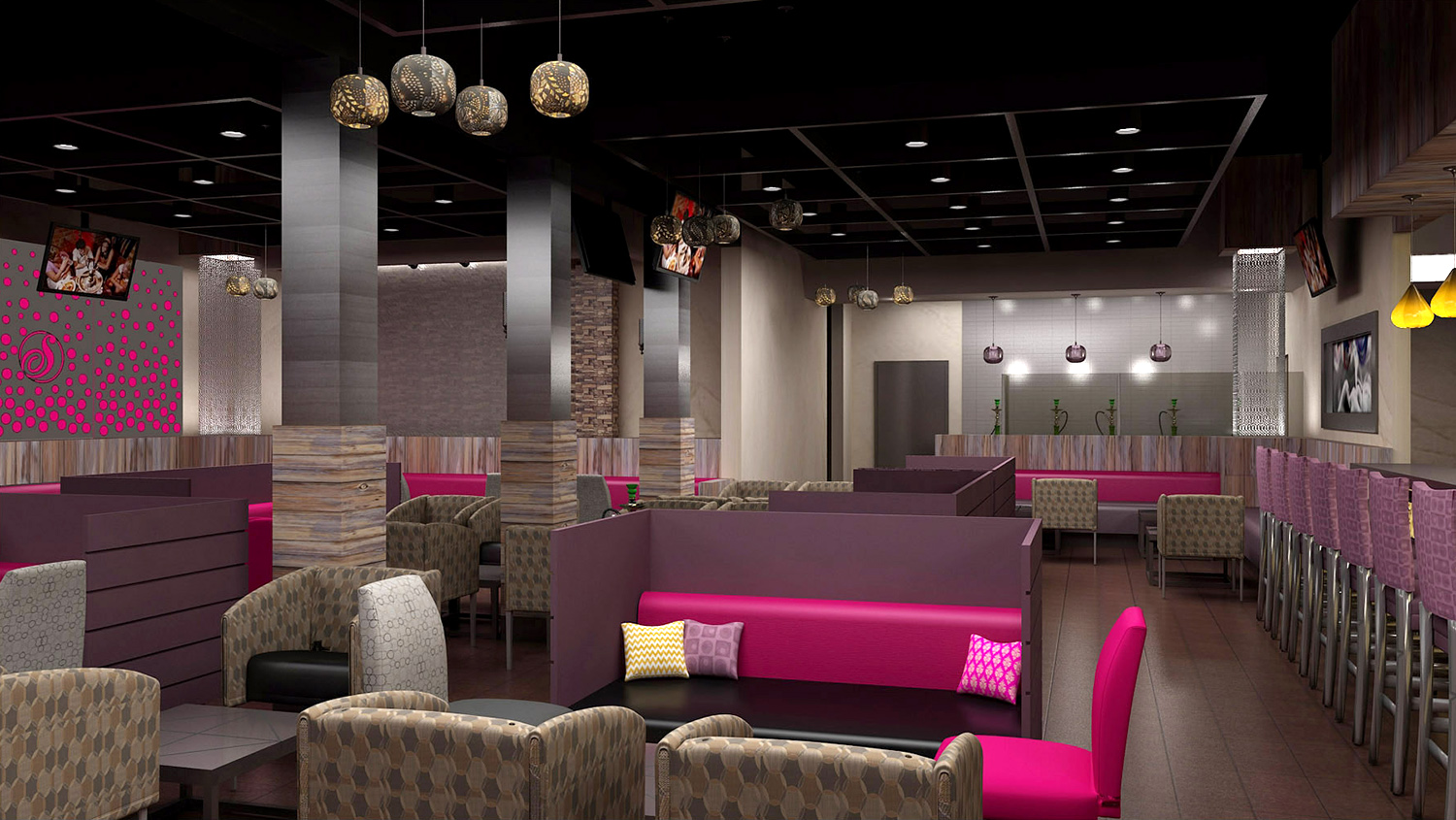The image depicts a darkly lit room with a modern and clean interior, likely a restaurant or a video game area. The room features a mix of seating arrangements, including various cushioned fabric chairs with a beige and gray pattern, a central hot pink couch adorned with throw pillows, and a hot pink-backed chair. The left side of the room showcases gray walls with hot pink accents and a small TV mounted on one wall. Hanging from the ceiling are silver, ball-like lights, with additional embedded ceiling lights, particularly clustered in the top left corner. To the right, there is a counter with multiple bar stools that have purple backs. The wooden flooring complements the room's sleek design, and the prominent use of pink elements suggests it might be a signature color for the establishment. The overall ambience is clean and stylish, though no people are present in the scene.